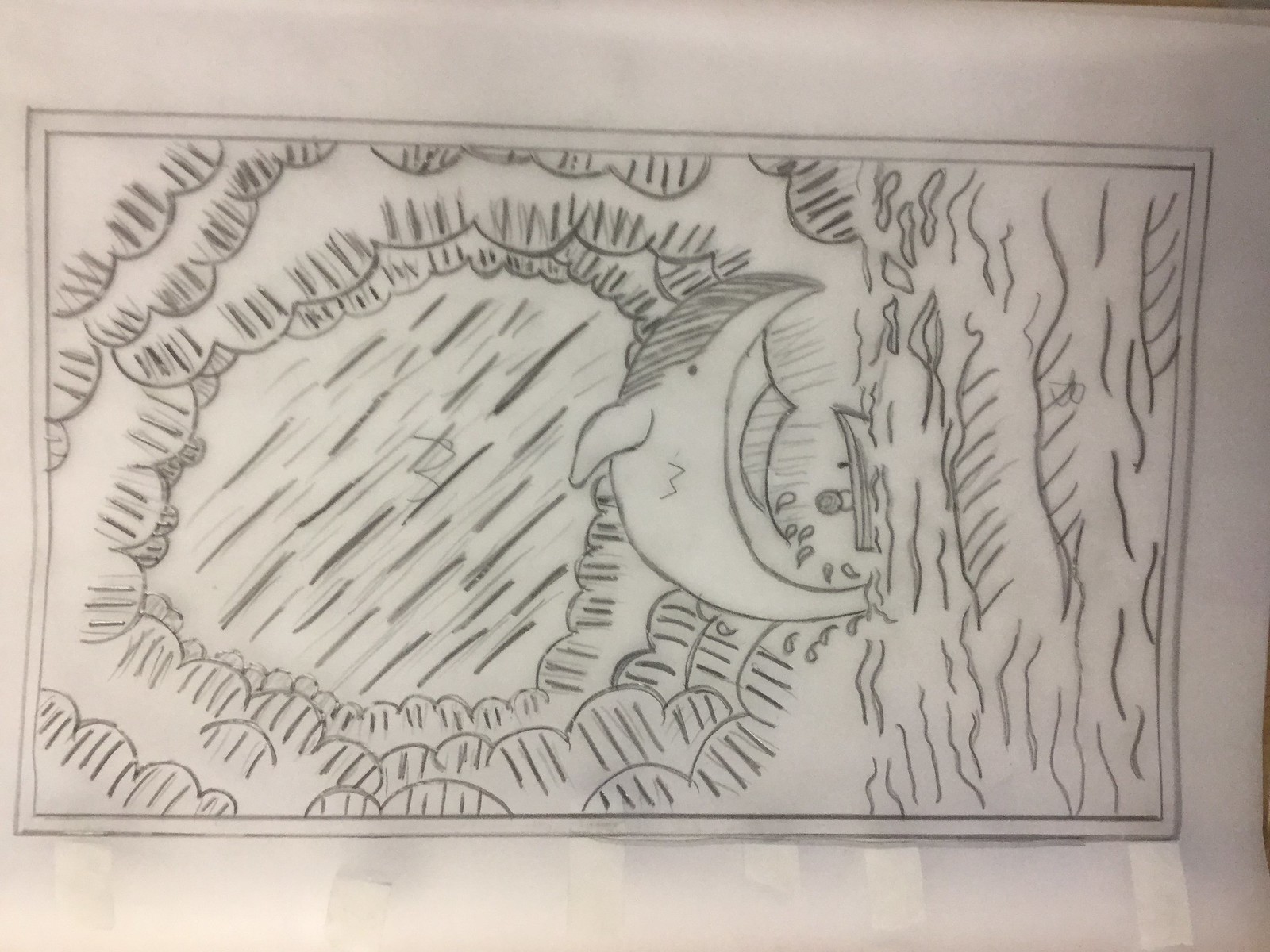This rectangular pencil sketch captures a mesmerizing scene of a diving porpoise emerging dramatically from the water. The meticulous shading on the porpoise's head and the surrounding water creates a vivid sense of movement and depth, making the waves appear to ripple energetically. Below the porpoise, a small boat with a single visible occupant—seen from the back—is dwarfed by the magnificent marine creature above. The person’s head peeks out from the boat, suggesting awe or contemplation as they gaze upwards. Adding to the ethereal quality of the artwork, the upper portion features a celestial, star-like whirl of clouds, layered intricately like the petals of a flower. This heavenly ambiance enhances the spiritual undertone of the scene, giving it an almost otherworldly feel as the porpoise appears poised to descend towards the boat.